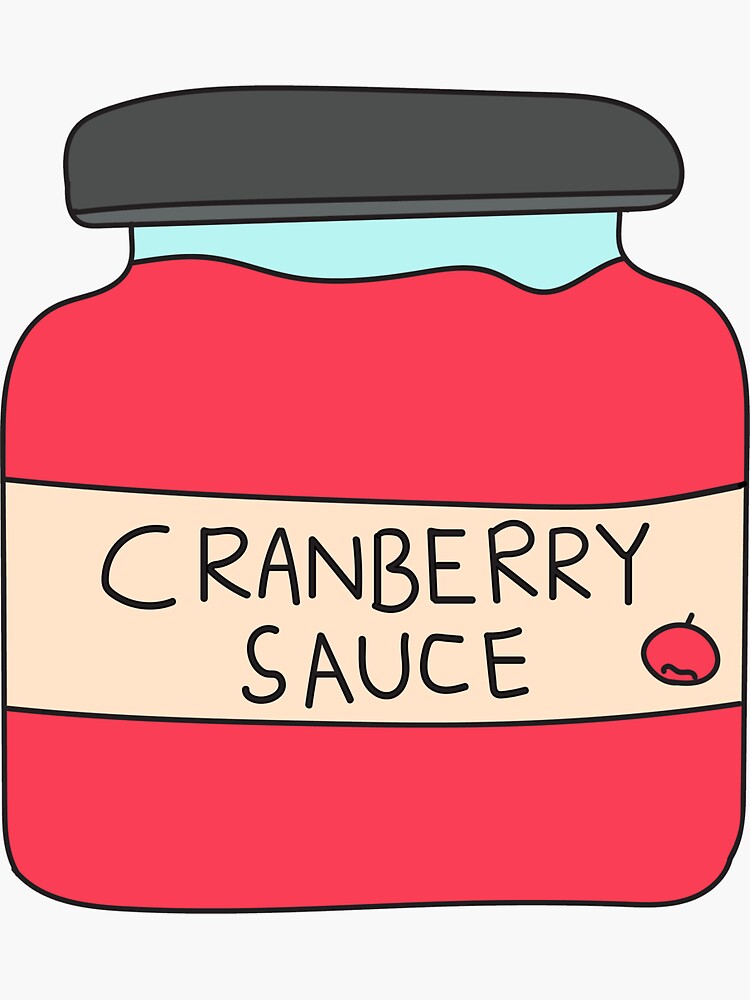This image features a hand-drawn, cartoon-style depiction of a jar of cranberry sauce. The jar, which is hand-held in size, has a distinctive square-shaped body and is filled to the top with vibrant red cranberry sauce. It is equipped with a dark grey or black cap. The jar displays a tan label that reads "cranberry sauce" in handwritten black lettering, accompanied by a small cartoonish drawing of a cranberry fruit. The entire illustration is set against a plain grey background, with no other elements present, making the cranberry sauce the sole focus of the image.